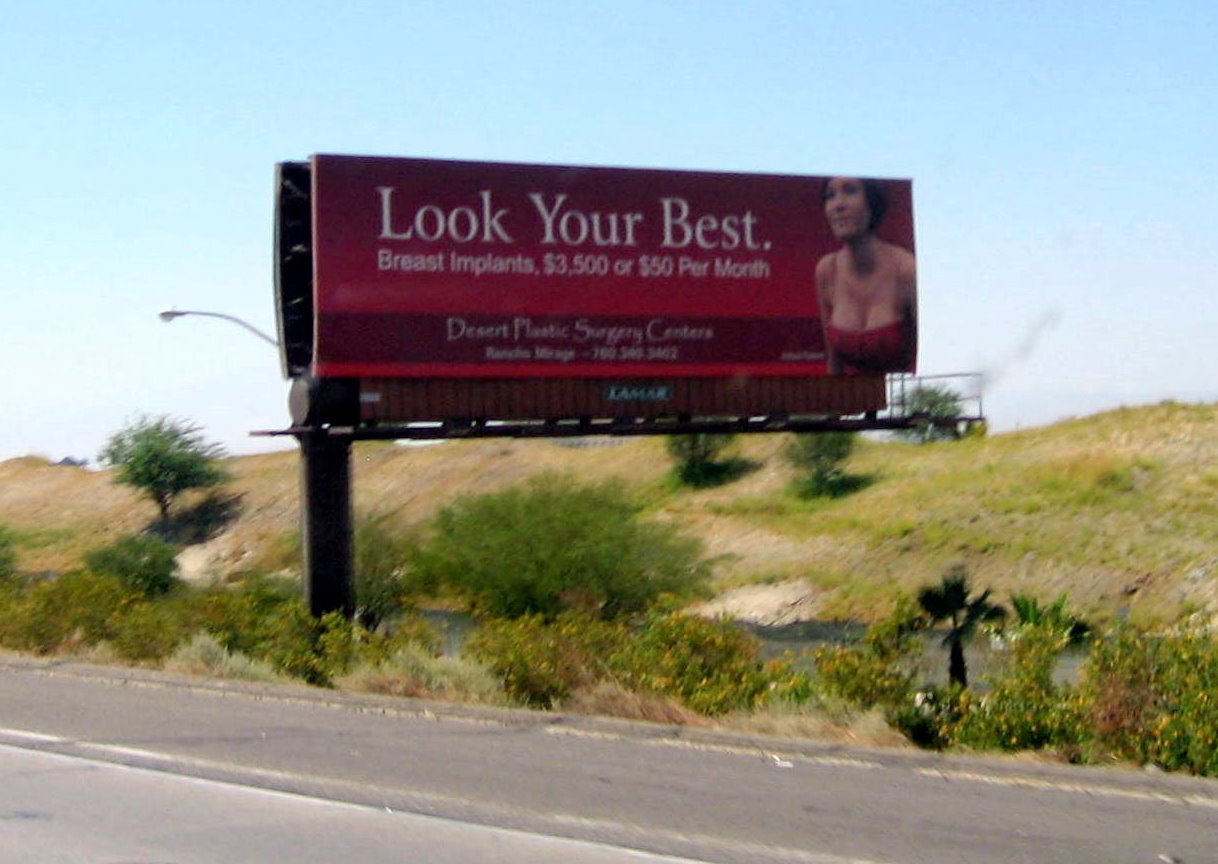Nestled on the side of a road, this scene showcases an incline dotted with large shrubs, patches of grass, and scattered rocks and boulders. A small strip of pavement is visible, leading the eye to a prominent red billboard directly ahead. The billboard features a vibrant red background and, in the right-hand corner, an image of an attractive, well-endowed woman with fair skin and short black hair. She is dressed in a strapless red dress. Bold, bright white text on the billboard advertises the "Look Your Best, Breast Plastic Surgery Center."